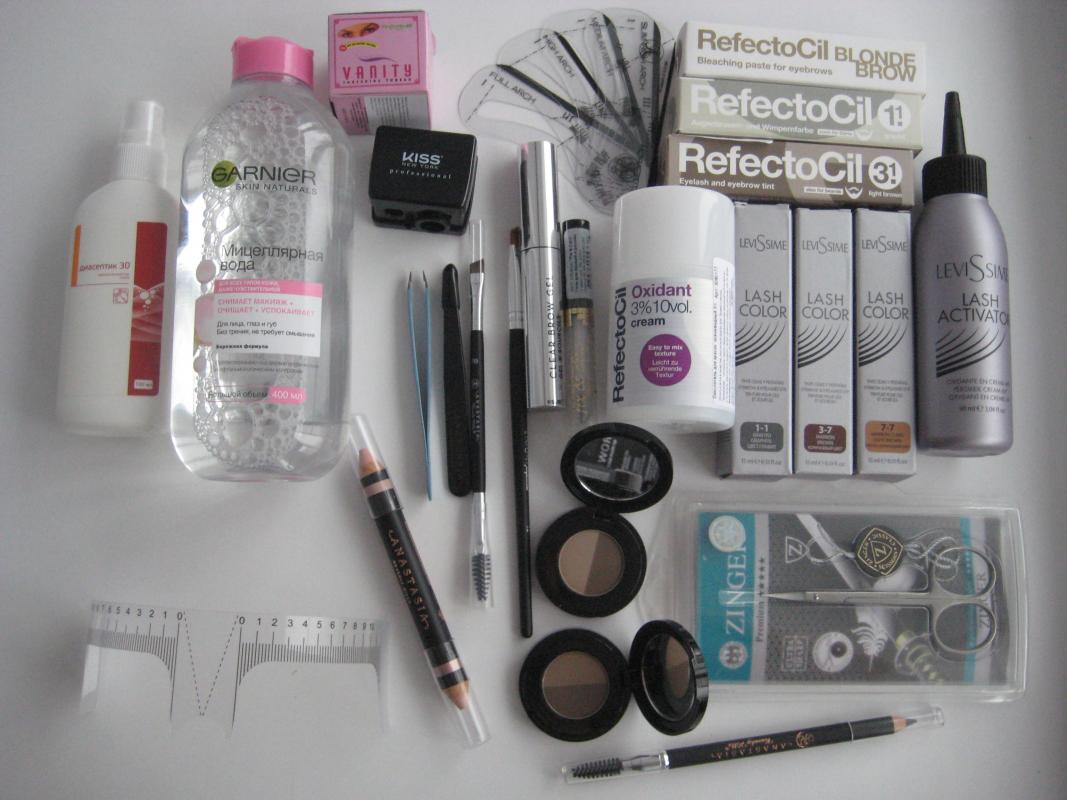A meticulously arranged assortment of personal care items dominates the frame, primarily featuring various makeup and skincare products tailored for women. On the left, two bottles stand out: a smaller, illegible white bottle, and a clear and pink bottle labeled in Russian, notable for being a product of the Garnier brand. Adjacent to these bottles are various face pencils or pens, accompanied by a precise pair of tweezers. 

The collection includes several types of brushes and a vibrant lipstick, hinting at an array of cosmetic applications. Scattered nearby are compact mirrors for on-the-go touch-ups. There's also a tube of oxidant cream, indicative of a more intensive skincare regimen. Three packages of eyebrow coloring kits are neatly aligned, flanked by boxes of lash color. Completing this extensive collection is a bottle of lash activator, a small pair of precision scissors, and another multi-purpose pencil at the bottom. The overall arrangement suggests a comprehensive toolkit for detailed and personalized beauty routines.